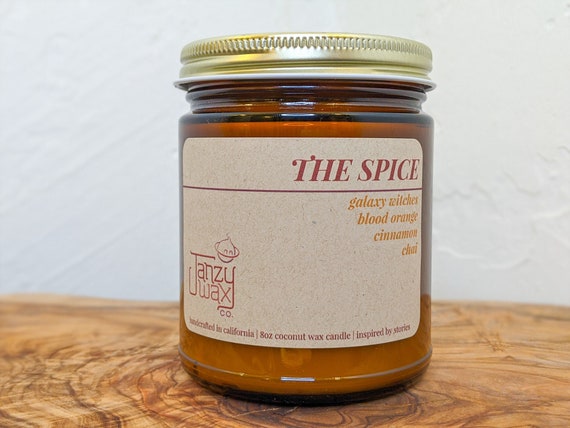This photograph captures an up-close view of a mustard-colored glass jar adorned with a brass screw-top lid. The jar, which contains an orange candle made from coconut wax, is positioned atop a brown wooden table with a plastered textured white wall in the background. The front of the jar features a detailed, beige textured label with bold and italic lettering. Prominently displayed are the words "The Spice Galaxy Widens," followed by "Blood Orange Cinnamon Chai" in bright orange and reddish-brown colors. The label also includes the name "Tansy Wax Company" accompanied by a logo of a round bomb with an orbit circle around it. At the base of the label, written in small lowercase letters, it reads, "Manufactured in California, 8-ounce coconut wax candle, inspired by stories." The overall composition and rich details emphasize the intricate design and aromatic theme of the candle.